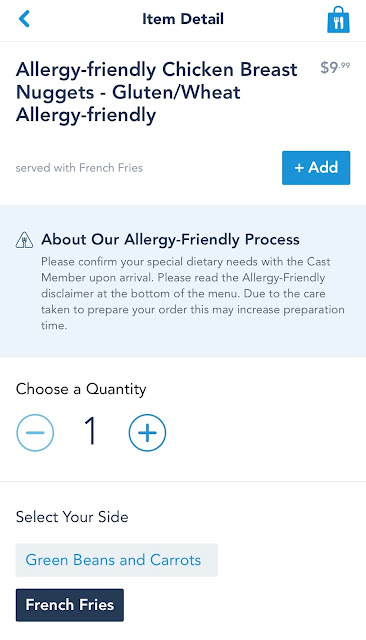To the right, there is a bag containing a stylish fork and an iron. Adjacent to it, a text block displays information about a dish titled "Allergy-Friendly Chicken Breast Nuggets - Gluten-Free - Sweet Allergy-Friendly," priced at $9.99. The dish is served with a side of french fries. Below that, a blue square features the label "Puss-Eyed."

Additionally, a gray square provides more details: "About our allergy-friendly process: Please confirm your special dietary needs with the cast member upon arrival. Please read the allergy-friendly disclaimer at the bottom of the menu. Due to the care taken to prepare your order, additional preparation time may be required."

Further down, a section labeled "Choose a Quantity" includes a minus button, the number one, and a plus button to adjust the order quantity. Another prompt invites you to select a side, offering options such as green beans, carrots, and french fries. 

Lastly, the allergy-friendly nature of the "Chicken Breast Nuggets - Gluten-Free - Sweet Allergy-Friendly" dish is emphasized again, noting that the necessary care in its preparation may require extra time.